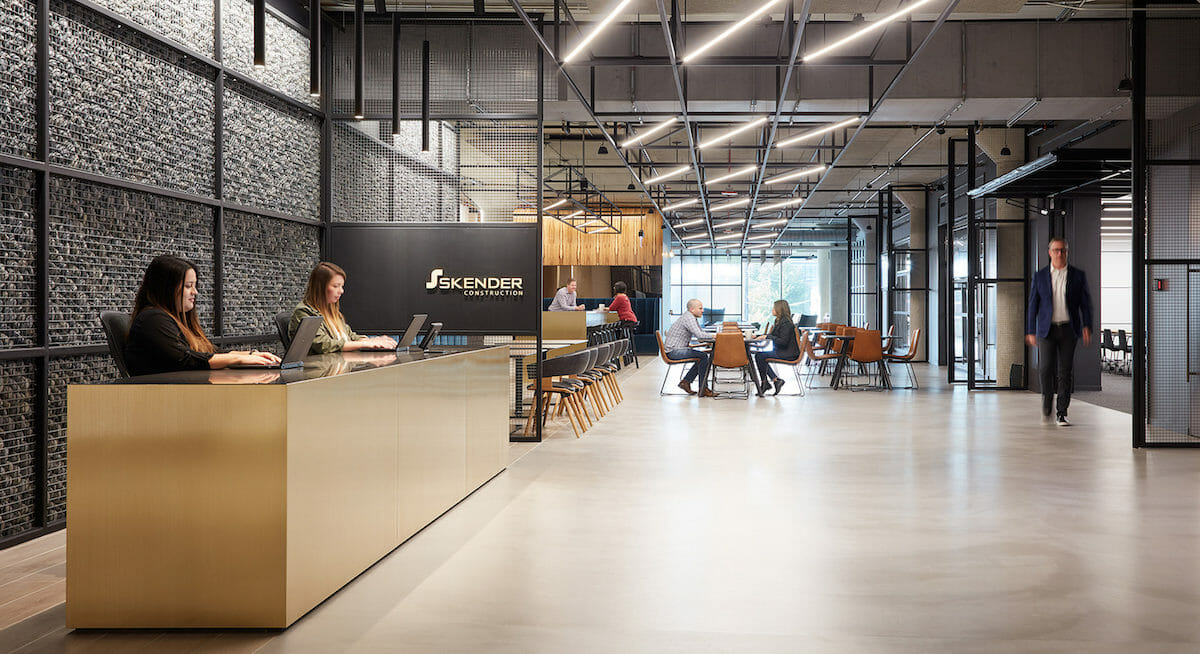The photograph depicts a modern reception area for Skender Construction, characterized by an exposed ceiling with gray metal bars extending up to a warehouse-style white metal finish. The walls to the left feature exposed gray brick with a metal frame. The reception area has a natural wood desk where two professionally dressed women with long hair sit, each working on a laptop. The company's logo, "Skender," is prominently displayed on a partial wall behind them. Beyond the reception desk, a man in a suit without a tie is walking past. In the spacious background is a meeting area with natural wood tables: a long table with two people sitting and conversing, and further back, a standing table with two more people in discussion. The area, filled with glass and elegant gray and brown tones, showcases a modern and well-designed environment.